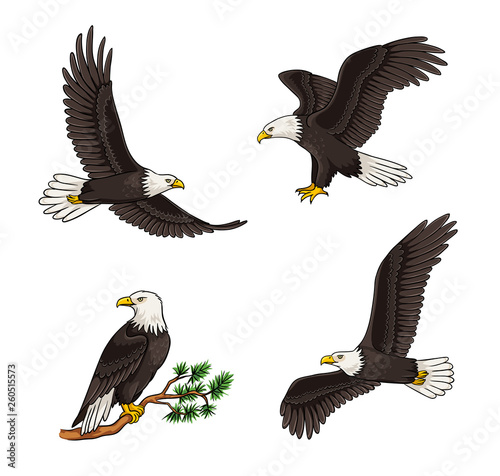The image is divided into four sections, each featuring a cartoonish, hand-drawn eagle in different poses, arranged in a window pane style with equal spacing. The top left section shows an eagle flying to the right with its legs trailing behind its tail. The top right section depicts an eagle landing with its wings outstretched and its feet extended as if grasping something. In the bottom left section, an eagle is perched on a branch, looking to the left, with some vegetation at the end of the branch. The bottom right section features another eagle flying to the left with its wings spread wide.

Covering the entire composition is a white semi-transparent watermark with the text "Adobe Stock" repeated diagonally across the image. Additionally, black text along the left edge of the image reads "Adobe Stock number 260-515573." The scene utilizes a color palette of white, brown, yellow, light brown, and several shades of green. The style is graphic and illustrative, resembling artwork that might be used on a website or purchased for use.